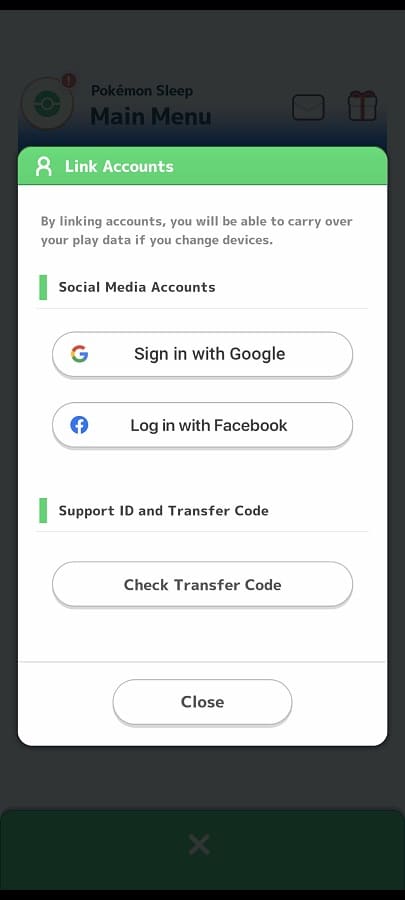A phone screenshot displaying a dark-tinted background page with partial visibility of menu items including "Sleep," "Main Menu," and a circular notification icon with a "Get" symbol. Dominating the screen is a pop-up window featuring a green-bordered header reading "Link Accounts" against a white background. The pop-up message informs users that linking accounts allows the carry-over of play data across devices. Below this message is an option to link social media accounts, with a prominent "Sign in with Google" button followed by a "Log in with Facebook" button. Further down, options for retrieving a Support ID and Transfer Code are available. An oblong, gray-bordered button with white interior labeled "Check Transfer Code" is visible. Finally, at the bottom, a smaller button with a similar design reads "Close."